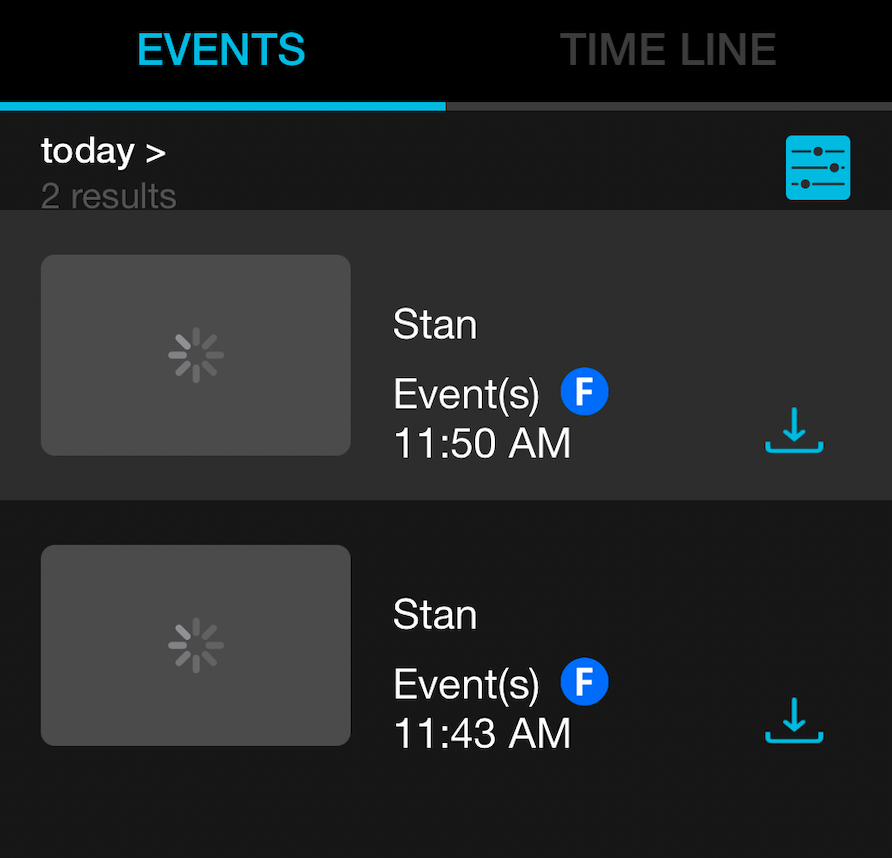The screenshot features a dark background. At the top left corner, "EVENTS" is displayed in light blue uppercase letters. On the top right corner, "TIMELINE" is shown in light gray uppercase letters. Beneath these headings, a horizontal gray line extends across the screen, with its left half highlighted in light blue.

Two lines below this, the word "TODAY" appears in white, accompanied by a right-pointing arrow. Directly beneath this, in gray text, the number "2" is followed by the word "results." Aligning with these elements on the right is an aqua blue square containing three horizontal black lines, each beginning and ending with a dot.

Below this section is a gray rectangle featuring a lighter gray rectangle on the left. Inside the lighter gray rectangle, a starburst-like symbol composed of multiple gray lines radiates from the center. To the right of this symbol, in white text, is the word "stand." 

Two lines down, the term "event(s)" is displayed in white, with the "S" placed in parentheses. Adjacent to this, there is a light blue circle with a capital white "F" inside it. Below this, the time "11:50 AM" is indicated in uppercase letters. Further to the right, an aqua blue download icon is visible, represented by a downward-pointing arrow with a horizontal line topped by two short vertical lines.

Below this segment, another gray square featuring the starburst symbol is present. To its right, the word "stand" is displayed, followed again two lines down by "event(s)" with the "S" in parentheses. Next to this is another light blue circle with a white capital "F." Below this, the time "11:43 AM" is indicated, followed by the same aqua blue download icon.